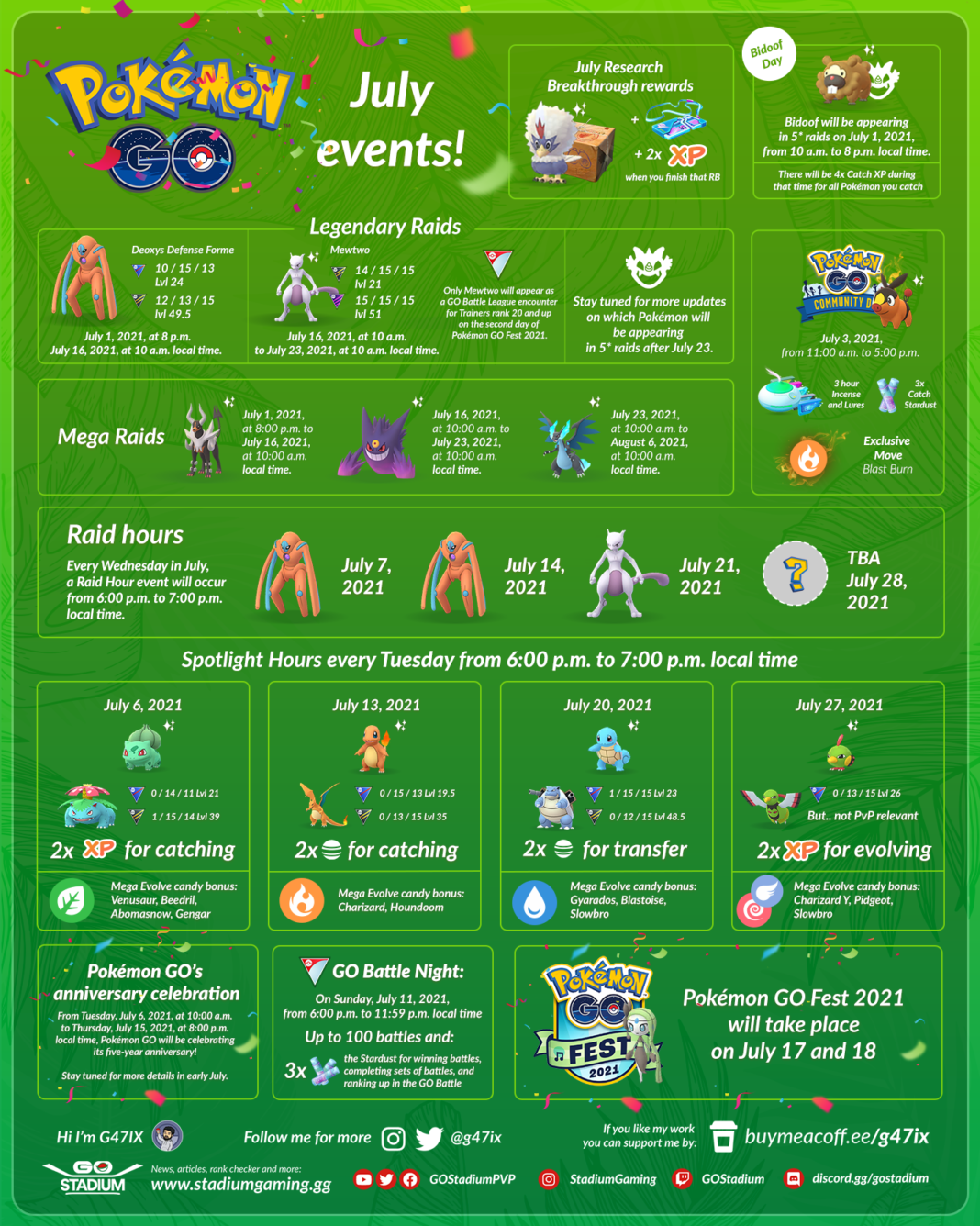This vertically-oriented image serves as a detailed calendar for Pokémon GO events in July. The background features a light green border, with an inner pea green section divided by a thin green line. The calendar's various segments are organized within neatly outlined green boxes, each containing specific event details.

At the top left corner, colorful confetti cascades down as a cheerful decoration. Beneath this, the bold heading reads "Pokémon GO" in blue text, with "July Events" in white just below it. To the right of these headers are details for each event:

- **July Research Breakthrough Awards**: An icon alongside the text indicates an additional two times the XP when completing the Research Breakthrough (RB).
- **Bidoof Day**: Features an illustration of Bidoof, highlighting its appearance on July 1st from 10 a.m. to 8 p.m.

Below these, the section is divided further:

- **Legendary Raids**: Listed with a white background, including relevant icons and information about the Legendary Pokémon available during the raids.
- **Mega Raids**: Information and icons display the Pokémon available for Mega Raids.
- **Raid Hours**: Specific times and dates for concentrated raid activities.

The image also addresses **Spotlight Hours** which occur every Tuesday from 6 p.m. to 7 p.m. local time, detailed with rewards for catching, transferring, or evolving Pokémon.

Additional sections include:

- **Anniversary Celebration**
- **Battle Nights**
- **Pokémon GO Fest 2021**: Scheduled for July 17th and 18th.

At the bottom, icons provide links to follow Pokémon GO on Twitter, Facebook, and Instagram, along with website URLs for more information.

This image serves as a comprehensive guide, detailing event dates, rewards, and participation opportunities for Pokémon GO enthusiasts throughout the month of July.